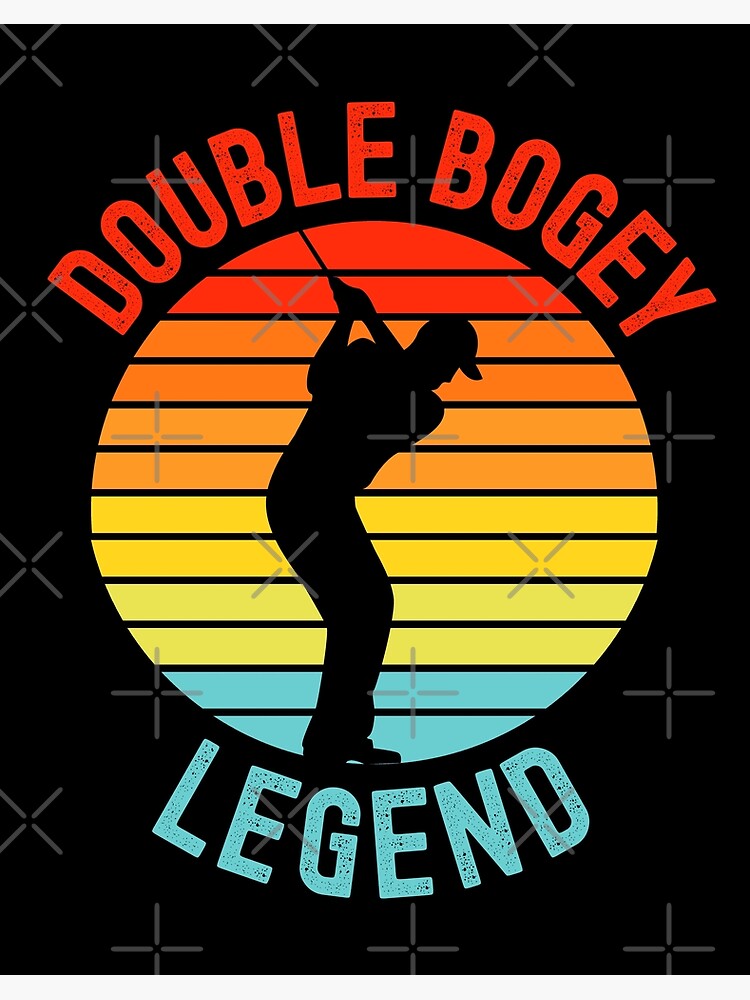The image depicts a black t-shirt or poster design featuring a striking graphic in its center. Dominant in the design is a black silhouette of a golfer, caught mid-backswing, with a golf club elevated over their shoulders. The golfer, bent at the waist and with knees slightly bent, wears a cap. This figure is encapsulated within a circular pattern resembling the sun, segmented into a gradient of colors: transitioning from red at the top, through various shades of orange and yellow, down to light blue at the bottom. Surrounding this central motif, the background is dotted with faint gray crosses and X-shapes, giving the impression of watermarks. Above the colorful circle, in bold red letters, is the phrase "Double Bogey," while below, in light blue letters, it reads "Legend," completing the vintage, meme-like aesthetic apt for a t-shirt or digital poster.